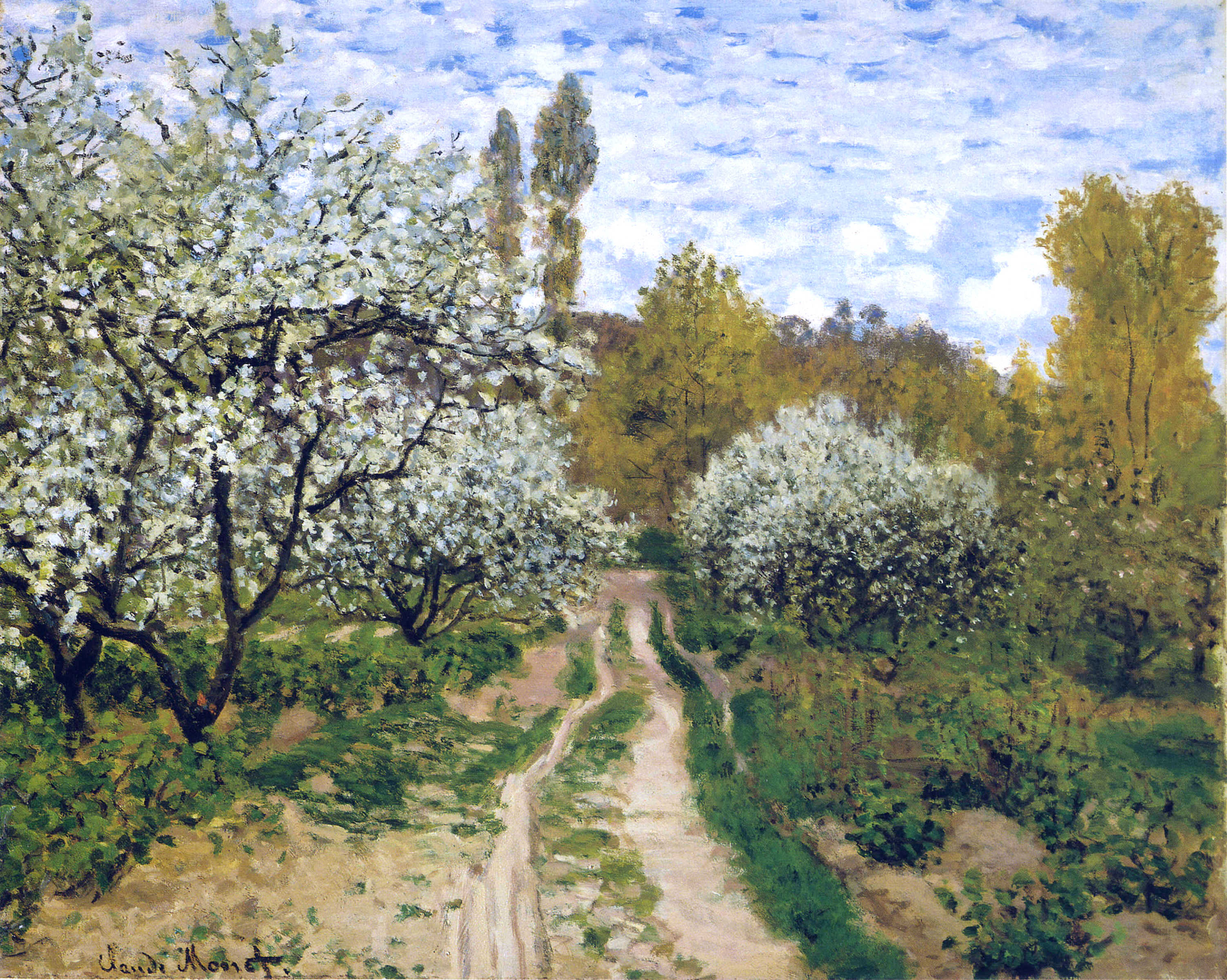The image is a detailed, realistic painting depicting a country scene under an overcast, cloudy blue sky with scattered white clouds. In the foreground, a dirt path extends upward from the bottom, framed by sections of grass in its middle, and flanked by dirt on each side. The path is bordered by various trees and bushes.

On the left side of the path, thin black-trunked trees with white, fluffy blooms, resembling cotton, stand prominently, with a couple more visible further down the path and into the distance. Similarly, on the right side, there are more of these trees alongside smaller bushes and grass. In the distance, the trees appear taller with green and yellow foliage, suggesting it is early fall with the leaves changing color.

The background reveals a variety of trees climbing up a slight hill, contributing depth to the scene. At the top, the sky is predominantly blue tainted with extensive white clouds, adding to the overcast ambiance.

Additionally, the lower left corner of the painting bears an inscription, potentially indicating the artist. The name appears to be "Monet," suggesting this might be a work by the renowned painter Claude Monet.